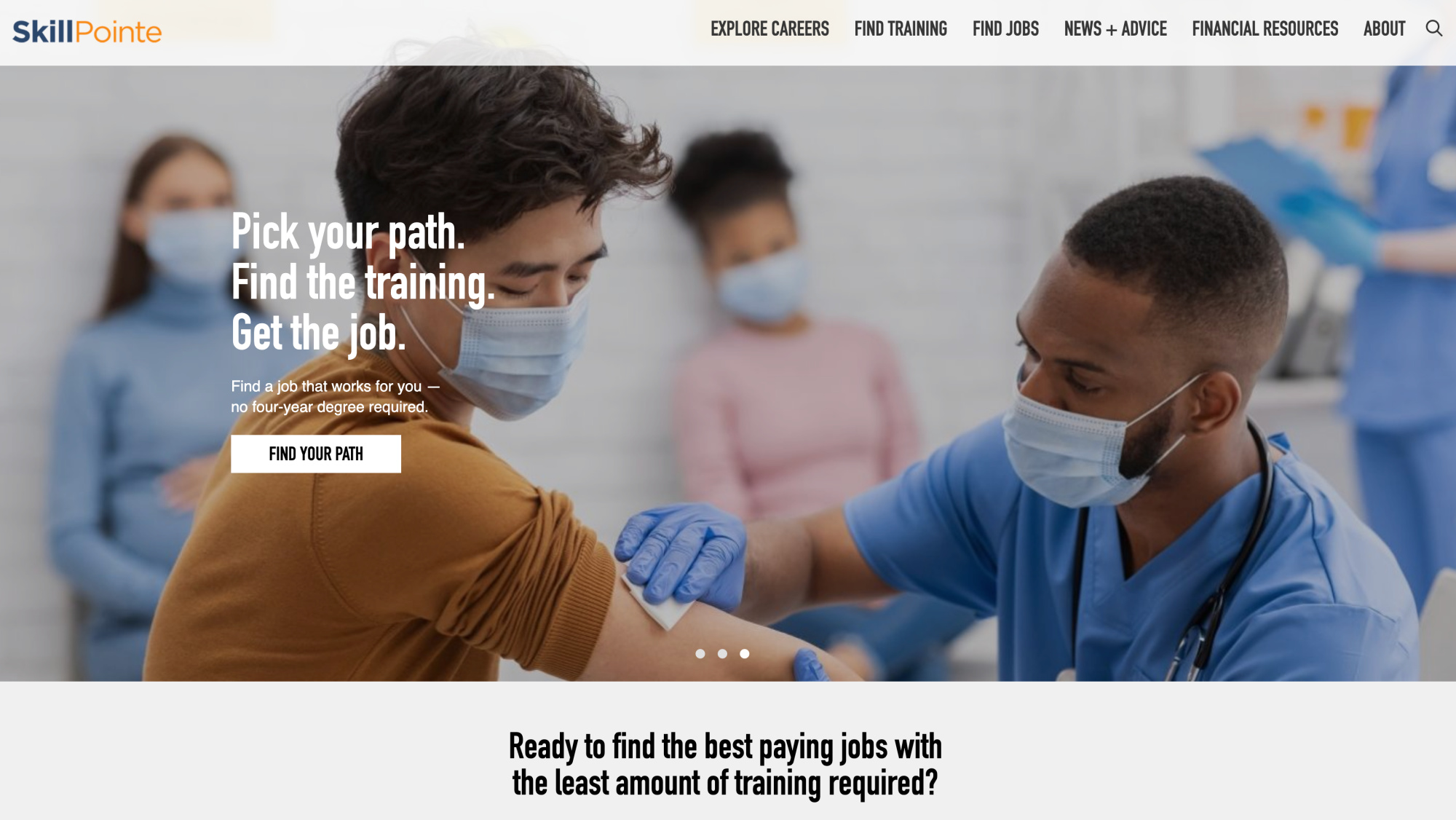The screenshot features the company logo "Skill Pointe" prominently displayed at the top. The word "Skill" appears in blue letters, while "Pointe" is written in orange-yellow letters on a light gray background. To the right of the logo are several navigation tabs labeled: "Explore Careers," "Find Training," "Find Jobs," "News + Advice," "Financial Resources," and "About," alongside a magnifying glass icon.

Below the navigation pane, a succinct message reads: "Pick Your Path, Find Training, Get the Job. Find a job that works for you. No four-year degree required." Beneath this message is a clickable button labeled "Find Your Path."

The main part of the screenshot showcases an image of a healthcare setting. A nurse, presumed to be of African-American descent, is seen wearing a face mask, blue hospital overalls, and blue gloves. He is cleaning a patient's right arm, which is exposed by a rolled-up t-shirt sleeve, likely in preparation for an injection. The patient, also wearing a face mask, appears calm and composed.

Below this image, three dots are lined up side by side, indicating that this is likely the third of a series of screenshots. At the bottom, a bold statement queries: "Ready to Find the Best Paying Jobs with the Least Amount of Training Required?"